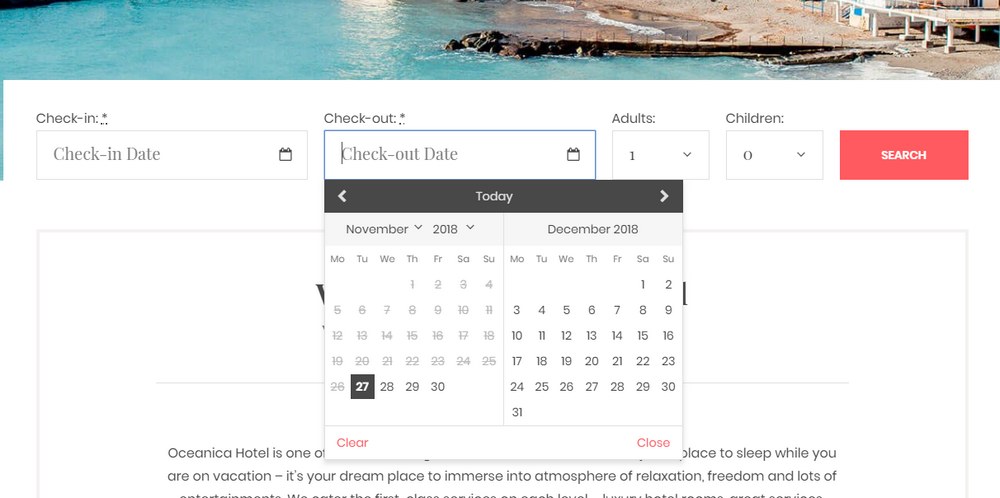The image appears to be a screenshot from a travel booking website, likely featuring a beach destination. At the top of the page, a banner partially obscured by a drop-down menu or pop-up spans across the screen. From what is visible, the background of the banner showcases a sandy area adjacent to vividly blue waters, possibly featuring a dock extending out into the water.

Directly below the banner, a user interface for selecting travel details is displayed. This section includes fields for "Check-in Date" which has an associated calendar icon. Beneath this, a drop-down menu is highlighted for "Check-out Date," showing today's date with available dates listed for November and December 2018. The selected check-out date is November 27th, 2018, indicated by a highlighted entry on the calendar. December 2018 currently shows no dates highlighted. Options to clear or close the calendar are provided in red at the bottom of the drop-down.

Further down the page, there are input boxes for the number of adults and children. The default selection shows one adult and zero children. Following this, there is a search bar for finalizing the search criteria.

The visible interface seems to pertain to booking at the Oceana Hotel, although the full description of the hotel is not readable due to it being blocked by the calendar drop-down. Despite the detailed interface, the name or branding of the booking site itself is not identifiable within the visible content of the image.